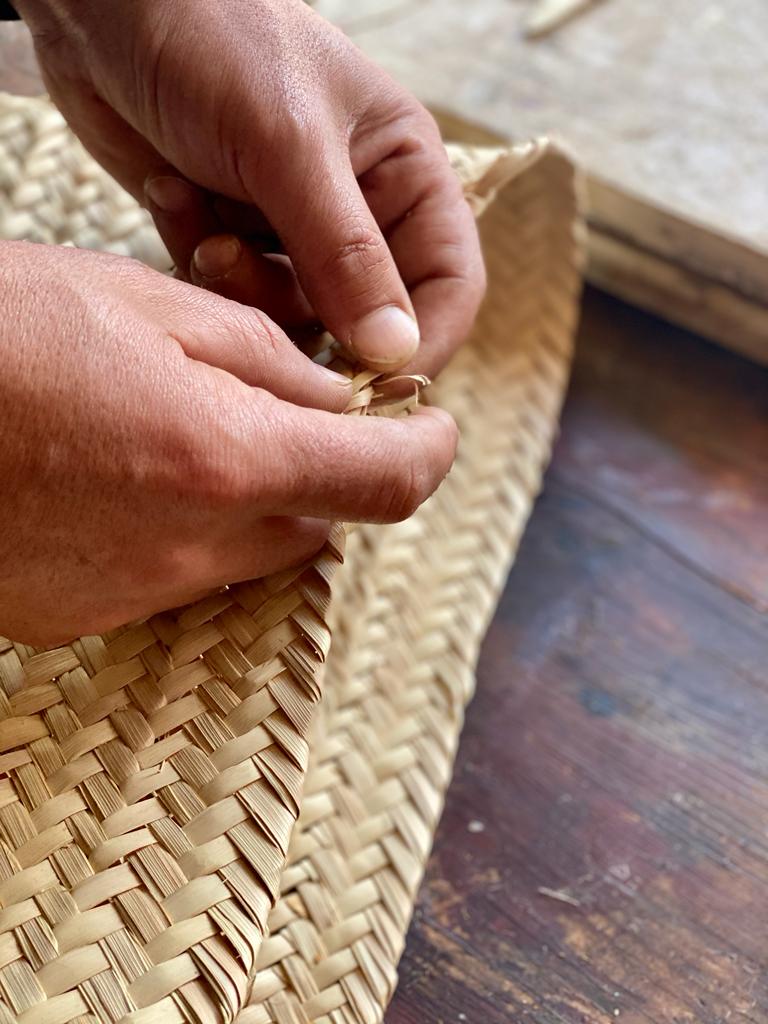The image features a close-up view of a female craftsman's hands meticulously weaving thin, tan-colored strips of material, likely flax or dried bamboo, into a basket. The scene is set on a wooden table covered with a red mat. The woven material starts at the bottom center of the image and extends in a folded pattern up and to the right, almost reaching the top before folding back down to the left. The craftsman’s right hand, positioned in the upper left section of the image, delicately threads the material, with the thumb and forefinger gripping one of the strips. The left hand enters from the upper left and supports the weaving process, with the fingers partially visible. In the upper right corner of the image, a white object is partially seen, and the right edge displays a dark wooden surface extending off the frame. The intricate craftsmanship and attention to detail highlight the process of creating a flexible, wicker-like basket.